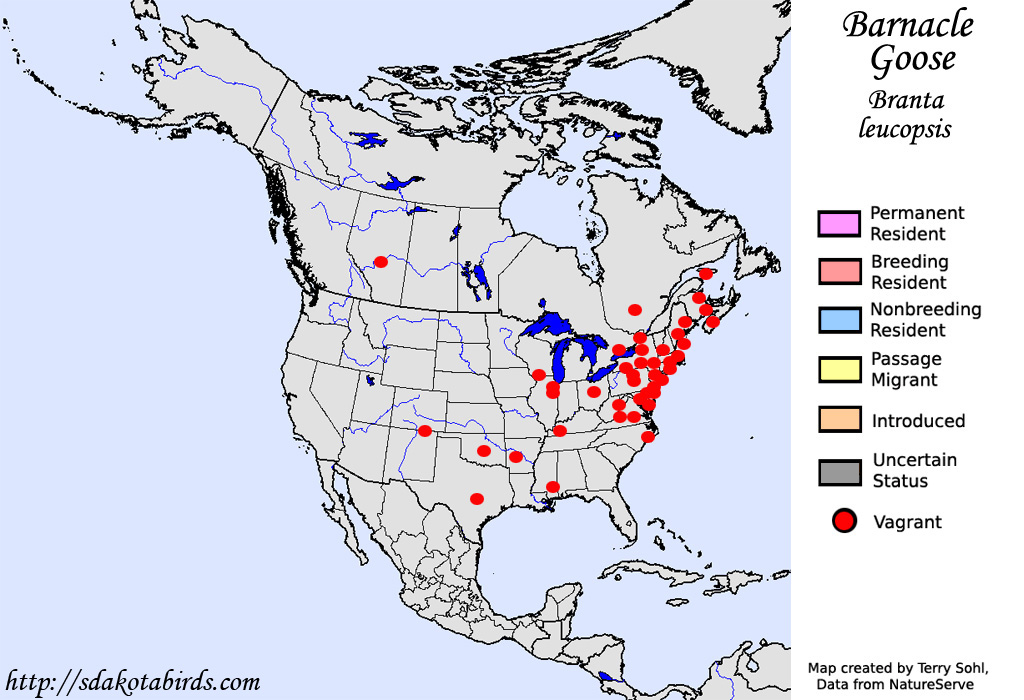The image is a rectangular map of North America, approximately six inches wide and four inches high. The right-hand side, starting about an inch from the upper right corner, features a plain white background with black text. At the top, it reads: "Barnacle Goose, Brontaleucopsis." Below this title is a legend in black print consisting of six colored rectangles and a red circle. These are labeled: permanent resident (light pink), breeding resident (pink), non-breeding resident (blue), passage migrant (yellow), introduced (peach), uncertain status (gray), and vagrant (red circle). 

The lower right corner of the white section states: "Map created by Terry Soule, data from NatureServe."

The left side of the image displays a map of North America, primarily in gray, highlighting different regions with small red circles concentrated in the Northeast United States, extending to areas such as Arizona, Texas, and Tennessee. There is minimal detail regarding state and city boundaries, and the background surrounding the map denotes the seas and oceans in blue.

In the lower-left corner of the image, the website "http://sdakotabirds.com" is printed in black text.